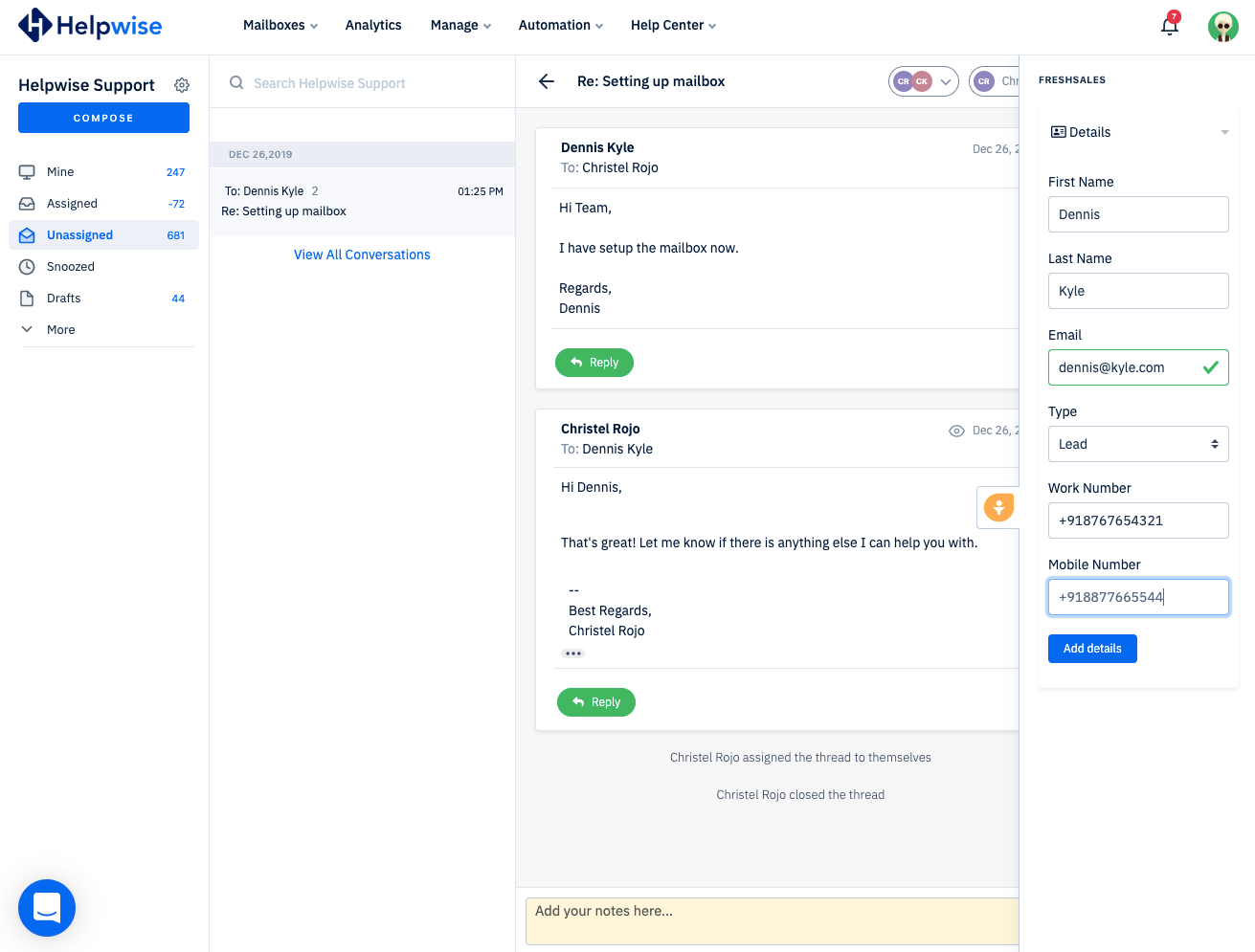**Caption:**

The image showcases the interface of Helpwise. At the top left, "Helpwise" is prominently displayed, followed by a navigation bar on the right featuring options such as "Mailboxes," "Analytics," "Manage," "Automation," and "Help Center." Below this, on the left side, the interface labels "Helpwise Support" next to a gear icon. 

A blue "Compose" button is situated underneath. Beneath this, several categories are listed: "Mine" with a count of 247, "Assigned" with a negative value of 72, and "Unassigned" highlighted in blue with a count of 681. Further down, there are options for "Snoozed," "Drafts" showing 44 items, and a "More" option. A blue icon resembling a speech bubble appears in the bottom left corner.

To the right, a search bar is labelled "Search Helpwise Support." Below, a conversation dated December 26, 2019, at 1:25 PM addressed to Dennis Kyle, under the subject "RE: Setting Up Mailbox," is displayed with an option to "View All Conversations." 

The conversation thread includes a message from Dennis Kyle to Crystal Rojo saying, "Hi team, I have set up the mailbox now. Regards, Dennis." Additionally, a green reply button is visible. Crystal Rojo's reply reads, "Hi Dennis, that's great, let me know if there's anything I can help you with. Best Regards, Crystal Rojo," accompanied by another green reply button.

At the bottom, a beige section prompts users to "Add Your Notes Here." On the right side, detailed contact information is presented, including "First Name: Dennis," "Last Name: Kyle," "Email: Dennis@Kyle.com," "Type: Lead," along with work, phone, and mobile numbers.